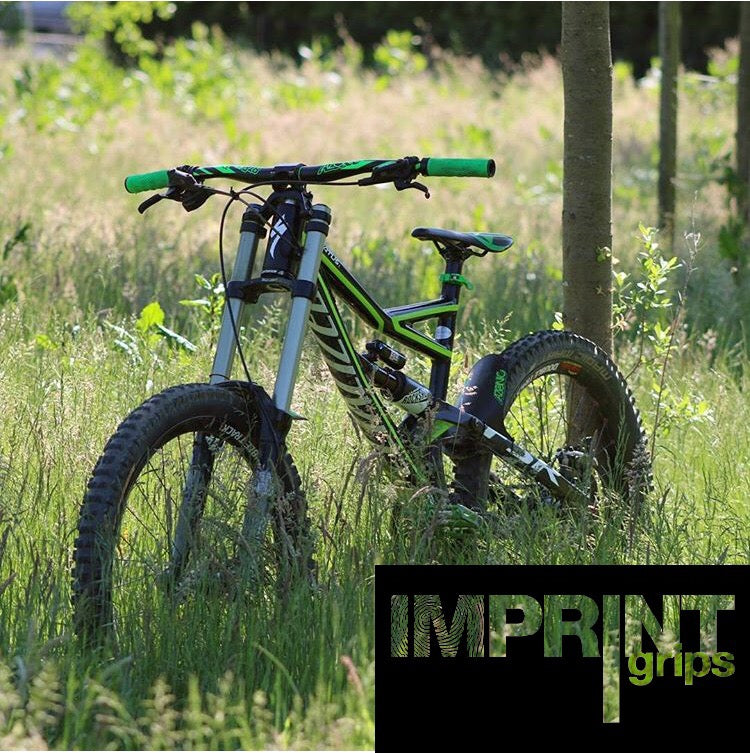This vertical photograph captures an outdoor scene dominated by tall grass, partially obscuring the bottom half of a vibrant green mountain bike. The bike is parked, leaning against a thin tree within a grassy field. The setting suggests a serene, possibly forested area, with the trunks of slender trees visible in the background. The bike itself features notable design elements including a green frame with neon green and black stripes, chrome front struts, thick black wheels, and green handlebars equipped with hand brakes. In the bottom right corner, the text "Imprint Grips" appears in a transparent font within a black square, indicating the brand or model of the bike. The overall atmosphere evokes a sense of tranquility and adventure, captured in a moment of stillness.